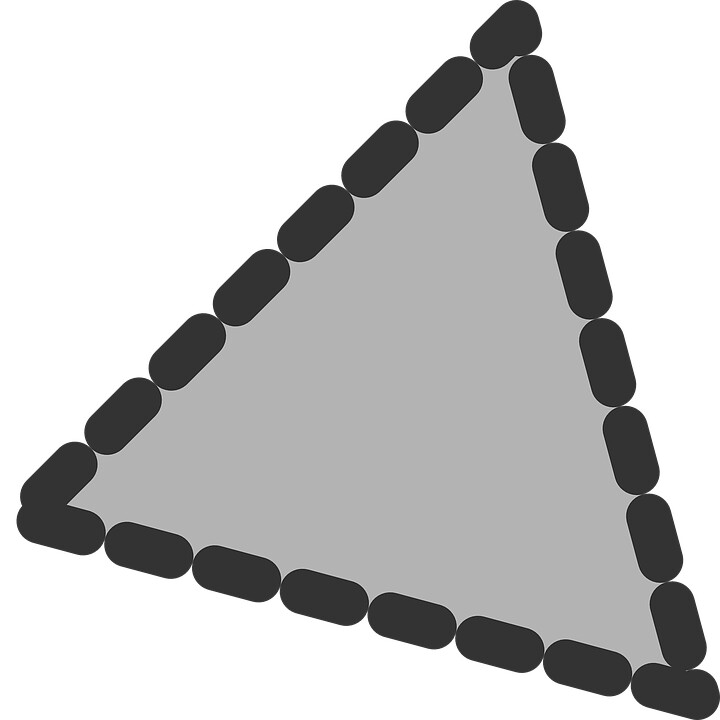The image features a large, gray triangle tilted to the right against a stark white background. The triangle is bordered by a continuous series of connected black capsules, resembling small, rounded pills or cocktail sausages, which create a distinct, cohesive outline. Each black capsule touches its neighbor without overlapping, forming a seamless perimeter around the gray triangle. The design's sharp contrast between the white background, the black capsules, and the gray interior of the triangle makes the image striking and visually compelling.